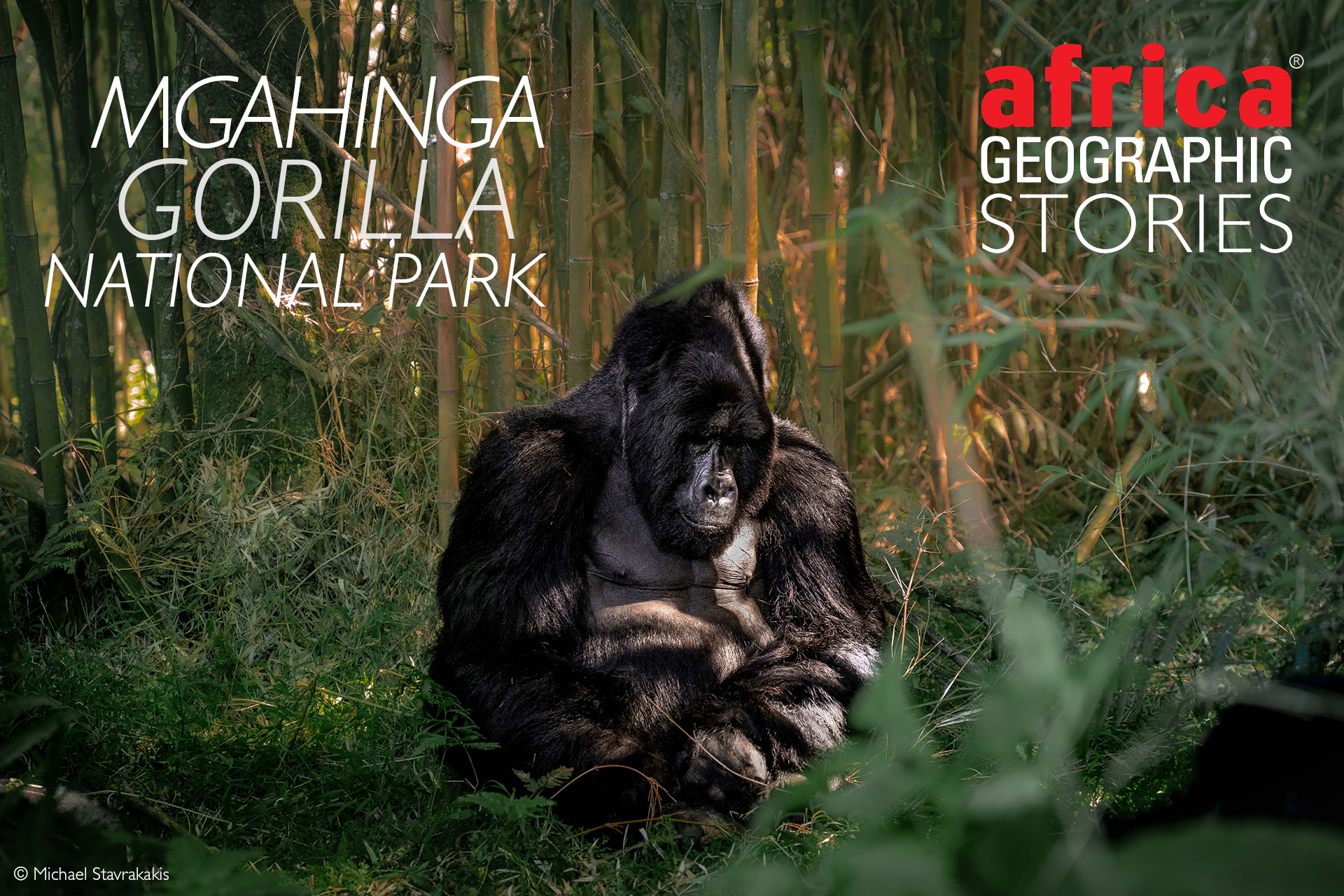The image is an advertisement for M-G-A-H-I-N-G-A (Mgahinga) Gorilla National Park. The poster prominently features a large, black gorilla sitting alone in the jungle. The gorilla appears to be at rest, with its thick, furry arms and legs crossed, and its massive head drooping down. The gorilla's face, chest, and nose area are covered in smooth, shiny black skin, creating a contrast with its dense fur.

Behind the gorilla, the lush jungle setting is vividly depicted, with green trees and bamboo shoots rising up, creating a canopy of greenery. The grass around the gorilla is dark and vibrant, contributing to the serene forest atmosphere.

In the upper right corner of the image, bold red text reads "Africa," followed by "Geographic Stories" in white letters, indicating a storytelling element. The upper left corner of the poster features the title "Mgahinga Gorilla National Park" in white letters. Additionally, the lower left corner includes a copyright notice with the name "Michael Staravicus."

The overall impression is one of peaceful solitude, with the gorilla appearing both majestic and somber in its natural habitat, surrounded by the dense and tranquil jungle foliage.